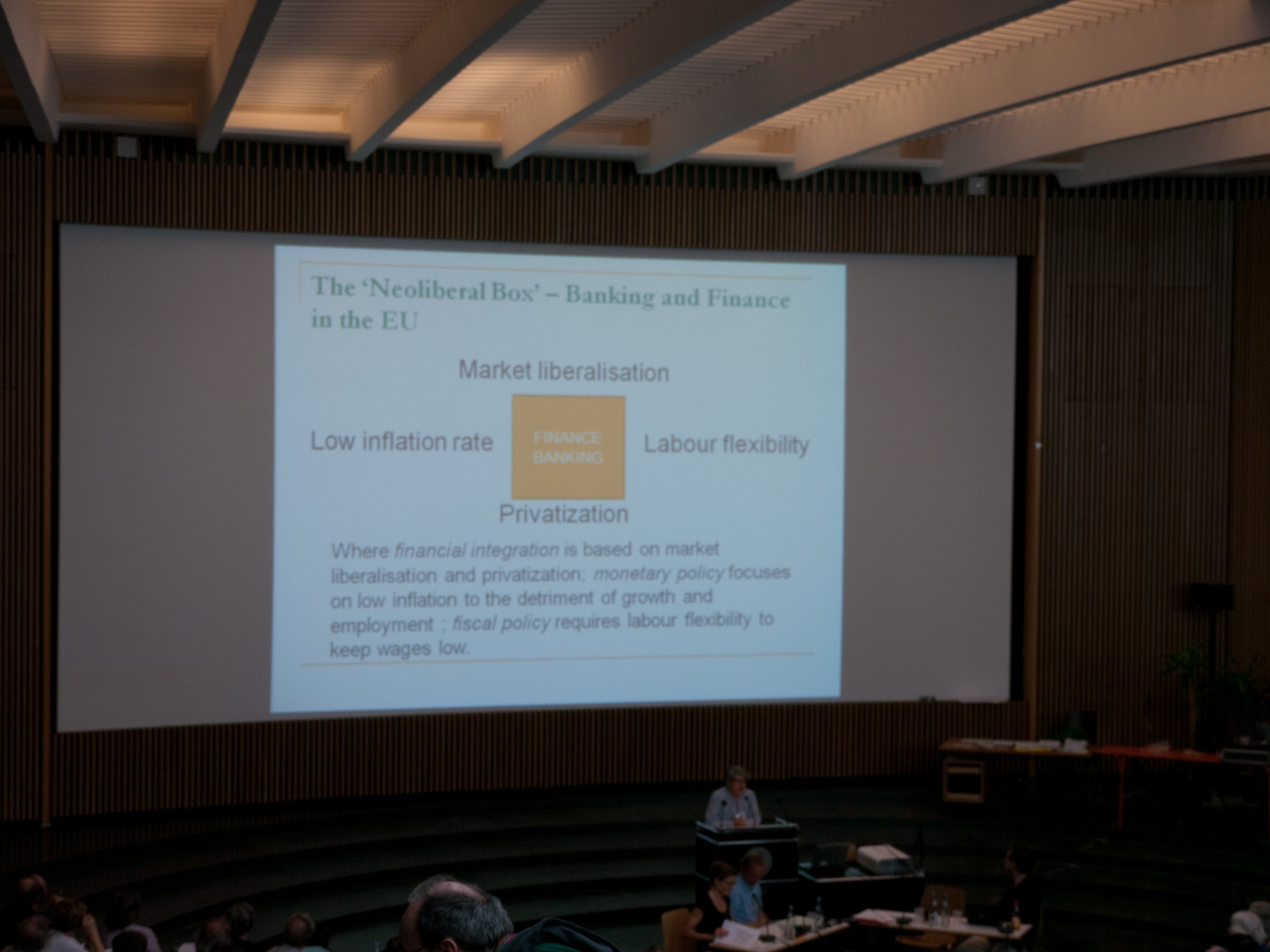The photograph captures an indoor conference hall or auditorium during a presentation or seminar. At the center of the image, an older woman stands at a podium, addressing a large audience with a microphone. She is slightly blurred due to the distance. Behind her, a massive screen displays a PowerPoint slide titled "The Neoliberal Box: Banking and Finance in the EU." Surrounding a central yellow square labeled "Finance Banking," the screen prominently features terms like "Market Liberalization," "Low Inflation Rate," "Labor Flexibility," and "Privatization." Below these keywords, a smaller paragraph reads: "Where financial integration is based on market liberalization and privatization, monetary policy focuses on low inflation to the detriment of growth and employment. Fiscal policy requires labor flexibility to keep wages low." In the foreground, several audience members, including a woman in a black shirt and a man in a blue shirt, are seated and attentively listening. The ceiling with visible rafters adds to the architectural detail. The overall ambiance suggests a formal and informative gathering.